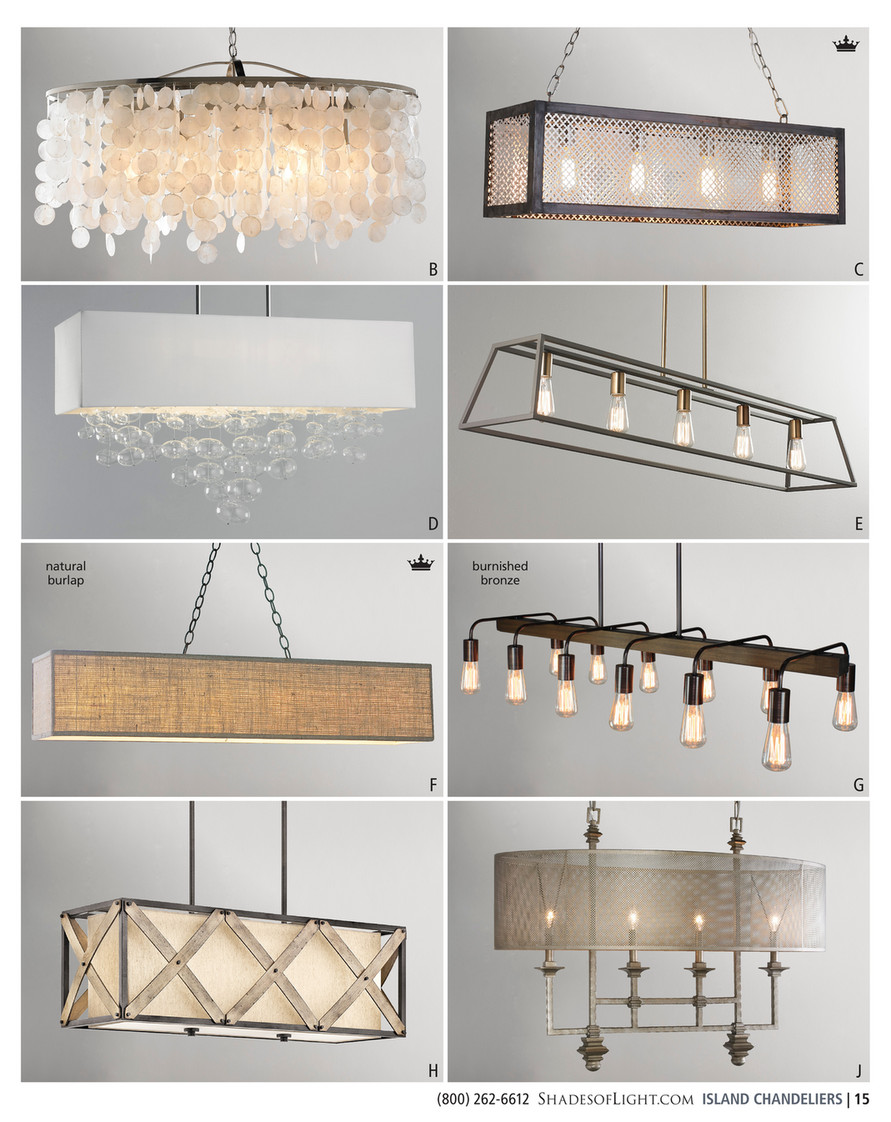The vertical rectangular image, styled as a catalog advertisement, features a collection of 8 modern-day chandeliers arranged in 4 rows and 2 columns against a grayish background. The top-left chandelier resembles cascading plastic snowflakes, creating a whimsical, wintery effect. Below it, a simple yet elegant plain white lampshade contrasts with the complex designs. Next is a chandelier with brown sides suspended by a chain, adding a rustic touch. The bottom fixture on this side is striking with silver X's and a black frame, supported by two posts.

On the other side, the first chandelier showcases transparent white circles hanging from the main structure, evoking an airy feel. Adjacent is a boxy design with grates on its sides, offering a peek at the lamps inside. The second row starts with a chandelier featuring a yellow rectangle adorned with bubble-like spheres. Next to it is a minimalist design with a rectangular frame holding five lamps. The third row begins with a chandelier resembling a paper box, emitting a soft glow. Following this is a linear piece of wood with lamps hanging beneath it, adding a natural element. Below is a rectangular box with decorative X's, and finally, the last chandelier in the fourth row is a sophisticated design with lamps that mimic the look of vintage candles, similar to candelabras found in a haunted mansion. At the bottom of the image, the advertisement text reads: "shadesoflight.com Island Chandeliers" followed by the contact number "800-262-6612".